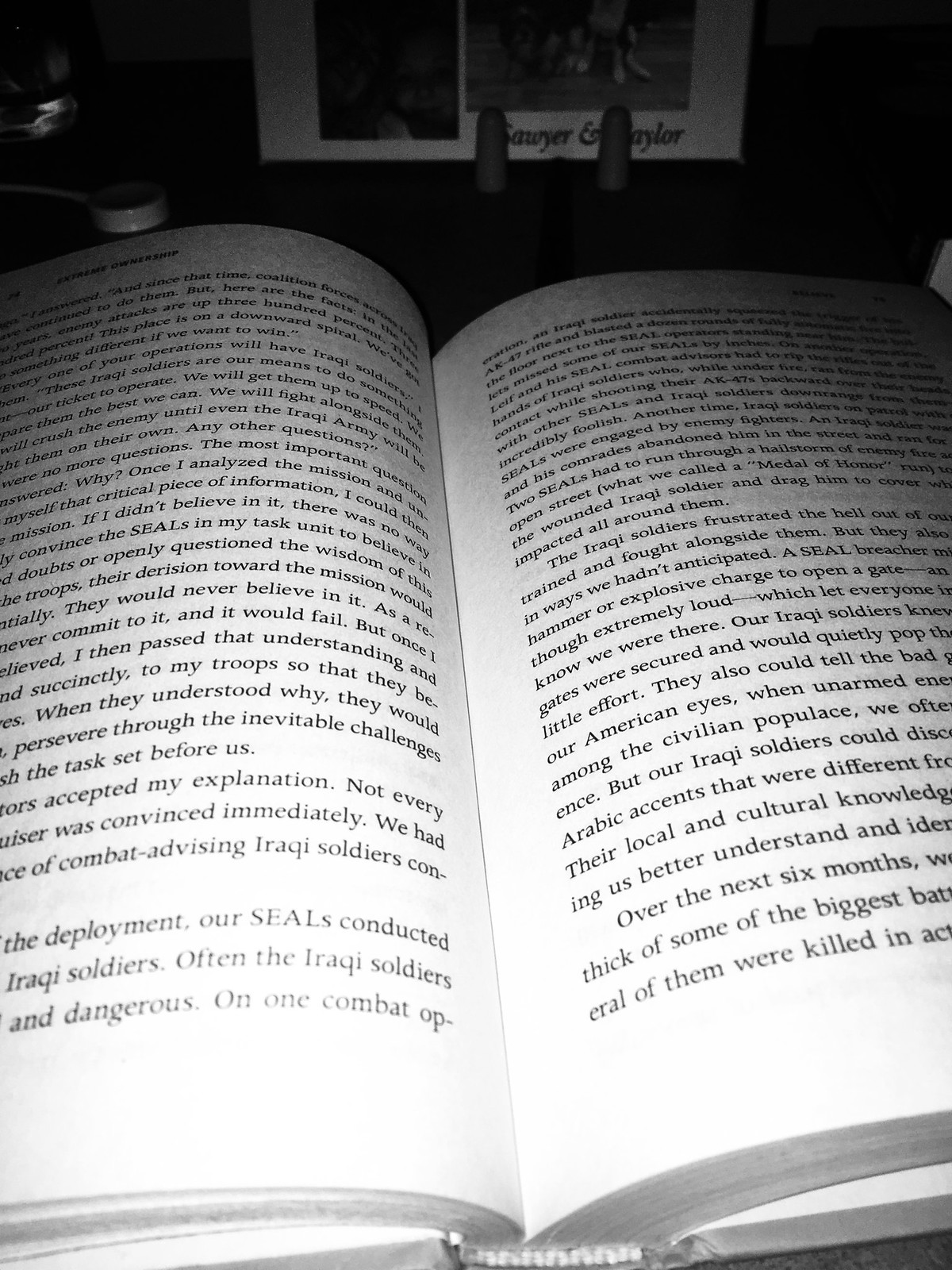The image features a close-up of an open book, likely centered beneath a light source aimed at the bottom of the pages. The book appears to be rather thick, indicated by the visible thickness at the bottom. The pages are white with black text, filled with a substantial amount of writing on both sides, suggesting the book is dense with information. Specific terms on the pages, such as "deployment our SEALs conducted," "Iraqi soldiers," and "local and cultural knowledge" suggest that the content focuses on Navy SEAL operations or military-related topics, although the complete context is unclear as only one page is visible.

A device, potentially a book holder, is used to keep the book open, with one arm of the device positioned in the upper center, contributing to holding the pages in place. In the background, there's a framed photograph of two people with the names "Sawyer" and "Taylor" written on it, partially obscured by the device. The background is fairly dark, adding contrast to the illuminated pages. Additionally, there are two elements resembling fingers sticking up in front of the photo, adding further texture and dimension to the scene.